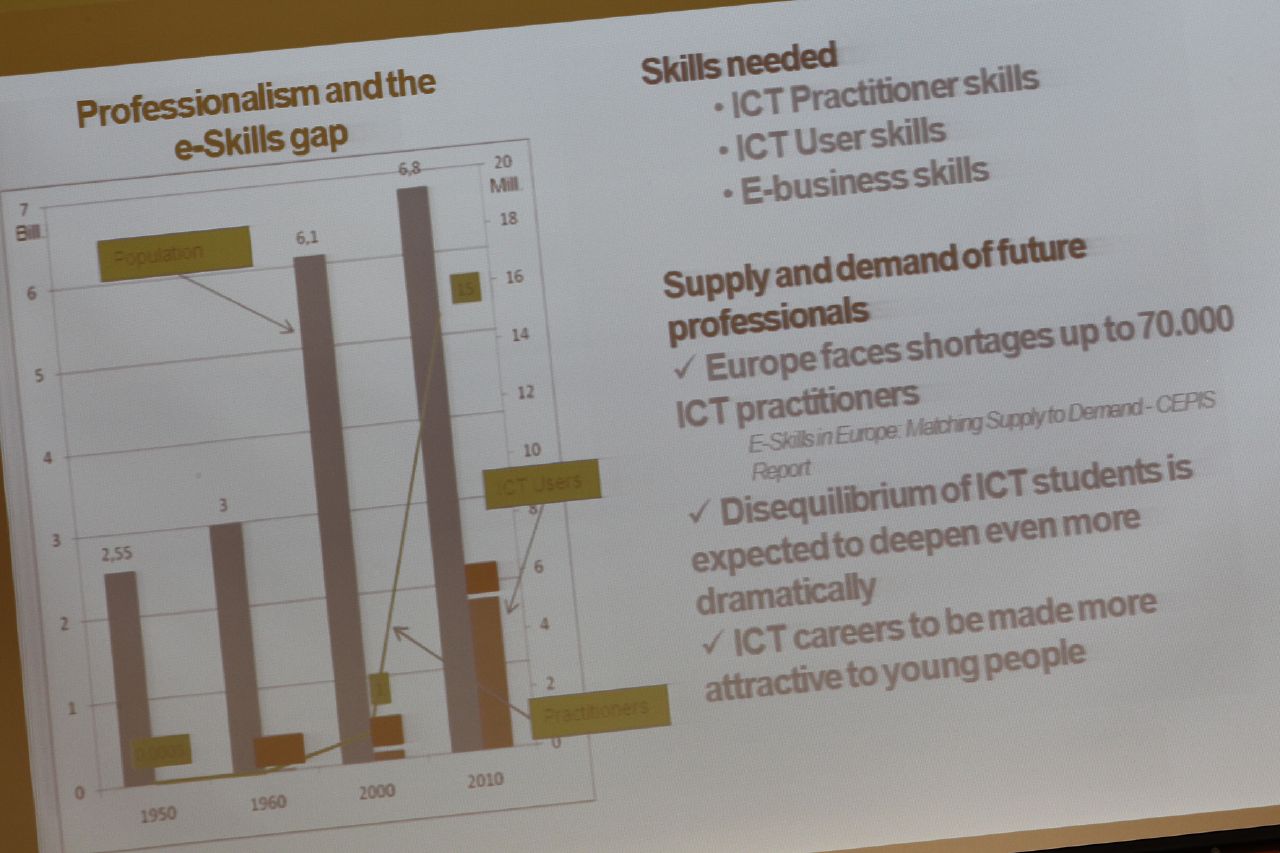The image showcases a detailed white informational poster mounted on a display stand. The heading, "Professionalism and the e-Skills Gap," is prominently displayed at the top in dark, bold letters. Below this, four vertical gray bar graphs represent data spanning from 1950 to 2010, depicting the population in millions. 

The bars increase in height from left to right, with the 1950 bar showing 2.55 million, 1960 at 3 million, 2000 at 6.1 million, and 2010 at 6.8 million. 

On the right side, in bold brown text, are the categories of skills needed:
- ICT Practitioner Skills
- ICT User Skills
- e-Business Skills 

Additionally, the poster details the supply and demand of future professionals, highlighting in bold brown that "Europe faces shortages of up to 70,000 ICT practitioners." A gray checkmark accompanies the statement, "ICT careers to be made more attractive to young people," underscoring the growing need for skilled professionals in the ICT field. The overall theme points to an increasing ICT skills gap and the anticipated deepening of this imbalance, presenting a call to action to attract younger individuals into ICT careers.